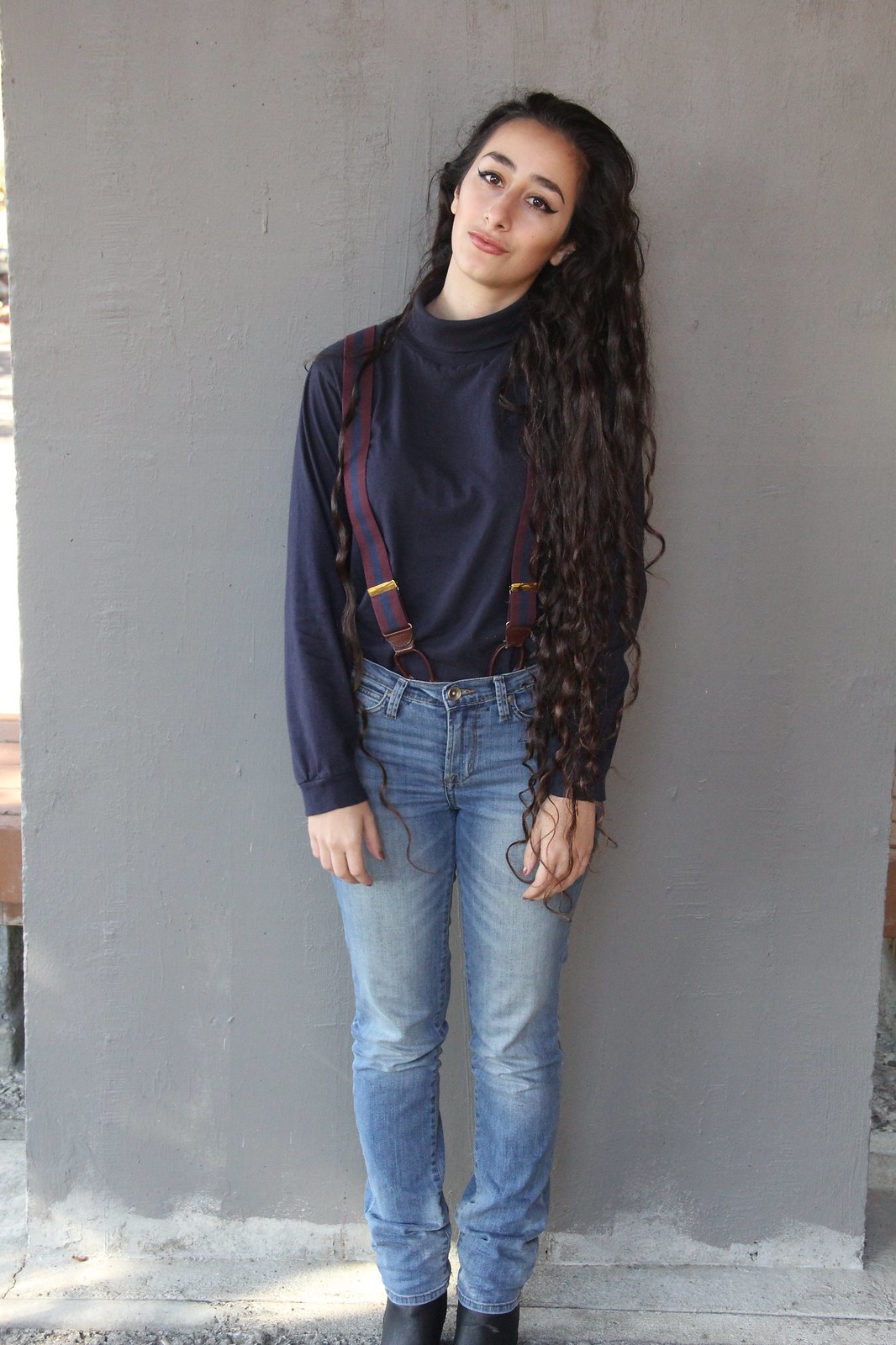In this image, we see a striking young woman, likely in her late teens to early 20s, standing against a partially painted, grey concrete wall that appears to be outdoors, with glimpses of sunlight and a sidewalk visible. She has very long, curly brown hair that cascades down to her thigh, partially covering her left shoulder while one strand rests on her right shoulder. Her complexion is light, and she has brown eyes. She could be Caucasian or possibly Hispanic or Persian. She is dressed in a navy blue, long-sleeved shirt, paired with navy blue and red striped suspenders attached to her somewhat tight-fitting blue jeans, and she wears black shoes. Her posture is relaxed, with her hands resting towards the front of her thighs, her head tilted to the right, and she looks directly at the camera with a neutral expression.